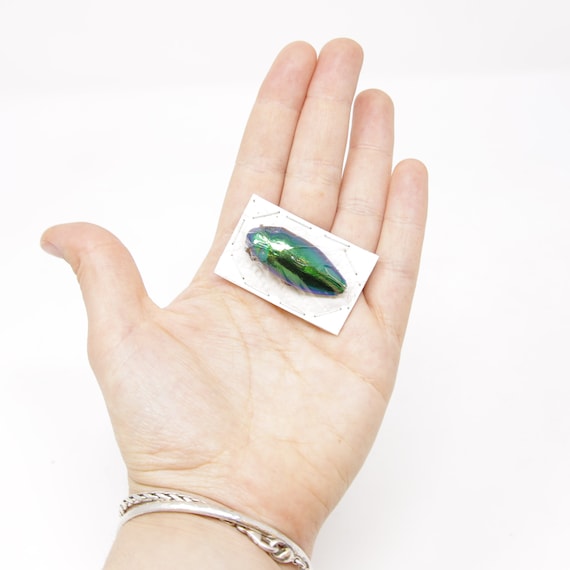In this vertically rectangular, full-color photograph, set against an off-white background, we see a close-up of what appears to be the left hand of a Caucasian woman. Her hand is positioned palm-up, with the wrist starting from the lower left and fingers pointing upward, slightly angled to the right. The thumb is extended outwards to the left. Resting in her open palm, near where the fingers connect, is a small, rectangular piece of white paper. On top of the paper lies a shiny green beetle, its shell reflecting light with hints of blue. The head of the beetle is oriented towards the left. The woman is wearing two wrist accessories: a smooth, probably silver or gold chain link bracelet, and a beige-colored hair tie that could be mistaken for a woven bracelet. The image appears to be taken indoors under artificial light, highlighting the vivid colors of the beetle and the neutral tones of the accessories.